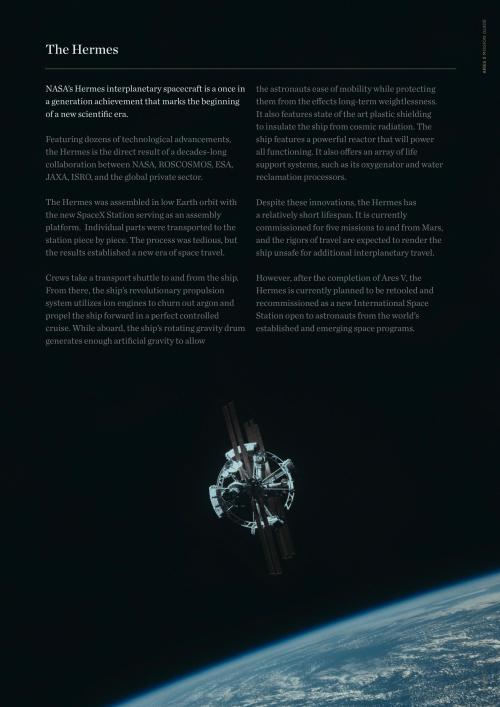A dark, star-studded outer space forms the backdrop of this evocative image. In the bottom right corner, the Earth appears as a distant blue marble amid the void. Dominating the center and extending slightly downward is a white, intricate structure—an orbiting satellite or space station, illuminated against the inky blackness. 

Overlaying this scene are seven distinct text elements, hinting at their importance through varying prominence. In the top left, a more conspicuous text reads "THE HERMES," standing out clearly against the dark expanse. Despite being less prominent, the words "NASA" and "that marks the beginning" are also visible among the other texts, written in a subdued gray, blending into the background of outer space. The overall composition juxtaposes the vast, silent universe with human technological achievement and exploration.